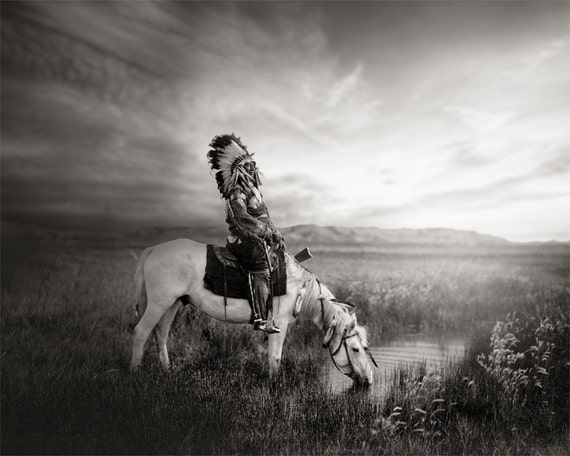The black-and-white image features a striking scene of a Native American man adorned in traditional clothing and a tall, feathered headdress, which adds a contrasting detail against the grayscale. He is mounted on a white horse that drinks from a pond in the foreground. Both the man and the horse are focused on, giving the background a slightly blurred effect, though it is evident that the expansive, grassy landscape is dotted with a few weeds on the right side. The horizon showcases imposing mountains, further emphasized by the clear sky, streaked with clouds that appear dark gray and white, creating a picturesque natural setting. The overall atmosphere suggests a serene, open area, possibly in the Midwest, with minimal vegetation beyond the grassy expanse.